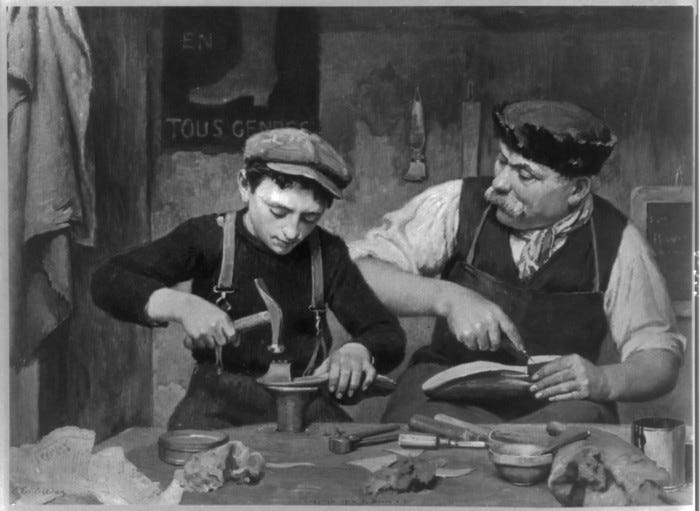This detailed black-and-white drawing, reminiscent of a lifelike print or oil painting, depicts an indoor cobbler's workshop setting. The square image features a thin gray border and presents a master cobbler and his apprentice at work, capturing an undeniable old-timey essence suggestive of the early 1900s or late 1800s. The older man on the right, distinguished by his bushy gray mustache, wears an apron and a dark cap with an upturned brim. He skillfully holds a boot, working on its heel with a specialized tool in his right hand while glancing attentively at the younger boy. The apprentice, dressed in suspenders and an old-style cap, focuses on hammering nails into the heel of an incomplete shoe. The workbench before them is scattered with various cobbling tools, materials, and rags, reflecting the meticulous and hands-on nature of their craft.